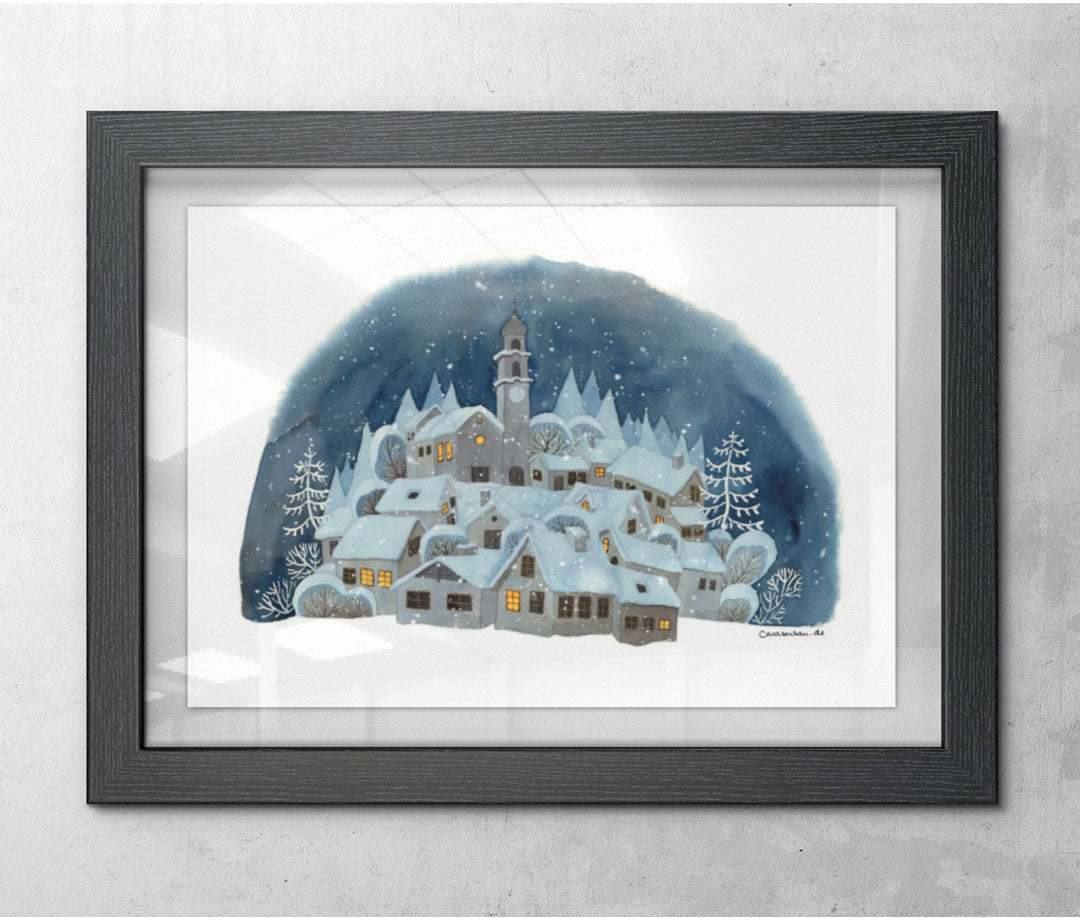The image presents a winter wonderland painting, possibly in oil, acrylic, or watercolor, framed in a plain black wood frame with a white mat border. The artwork encapsulates a serene, dome-like snow globe scene, featuring a quaint village perched on a hill. Snow is gently falling against a blackish-blue sky, blanketing the houses and landscape in pristine white. The village is comprised of multiple grey buildings, with yellow-lit windows adding a warm glow. Central to the composition is a prominent church with a steeple that stands atop the hill, flanked by smaller homes on descending tiers. Christmas trees and snowy foliage accentuate the idyllic scene, bringing a festive, cozy atmosphere to the tableau. The painting is signed at the bottom, lending an authentic touch to this enchanting depiction of a peaceful, wintery village.